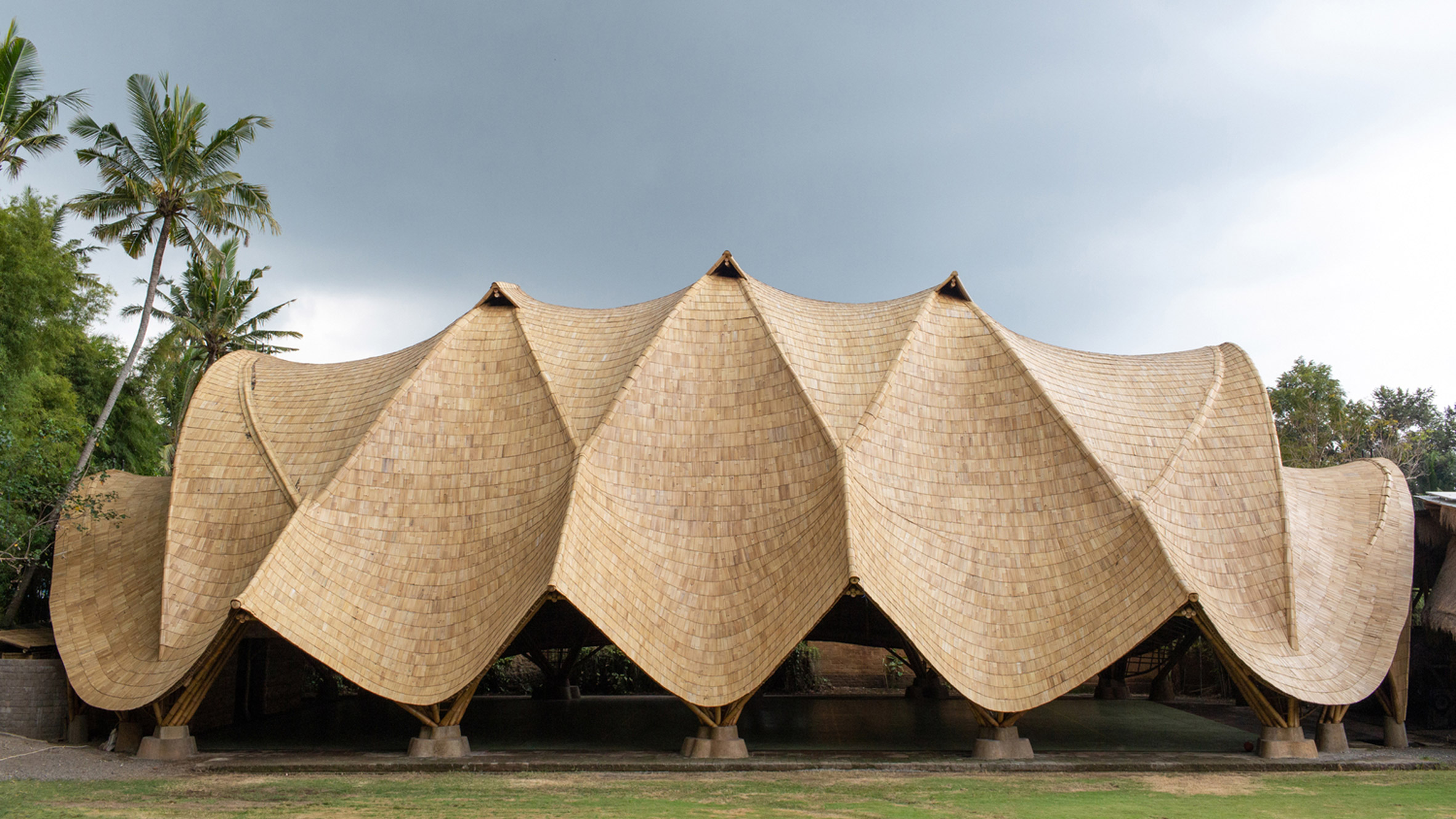This landscape photograph captures a fascinating Asian-inspired outdoor structure that resembles a traditional hut, possibly from Thailand. The structure is prominently tan, likely constructed from bamboo or a similar organic material, giving it an intricate, wavy design. The roof sweeps gracefully upward, mimicking mountain curves and forms pointed peaks that appear almost hat-like at the vertices. At the apex of these points, small openings can be seen, adding a sense of depth and shadow to the design. The structure stretches horizontally from the left to the right of the image, supported by vertical elements reminiscent of furniture legs, giving it a sense of stability despite its abstract shape. Surrounding the hut, there is a slim strip of grass in the foreground, and palm trees are visible on both sides, set against a cloudy sky that completes this exotic, tranquil scene.